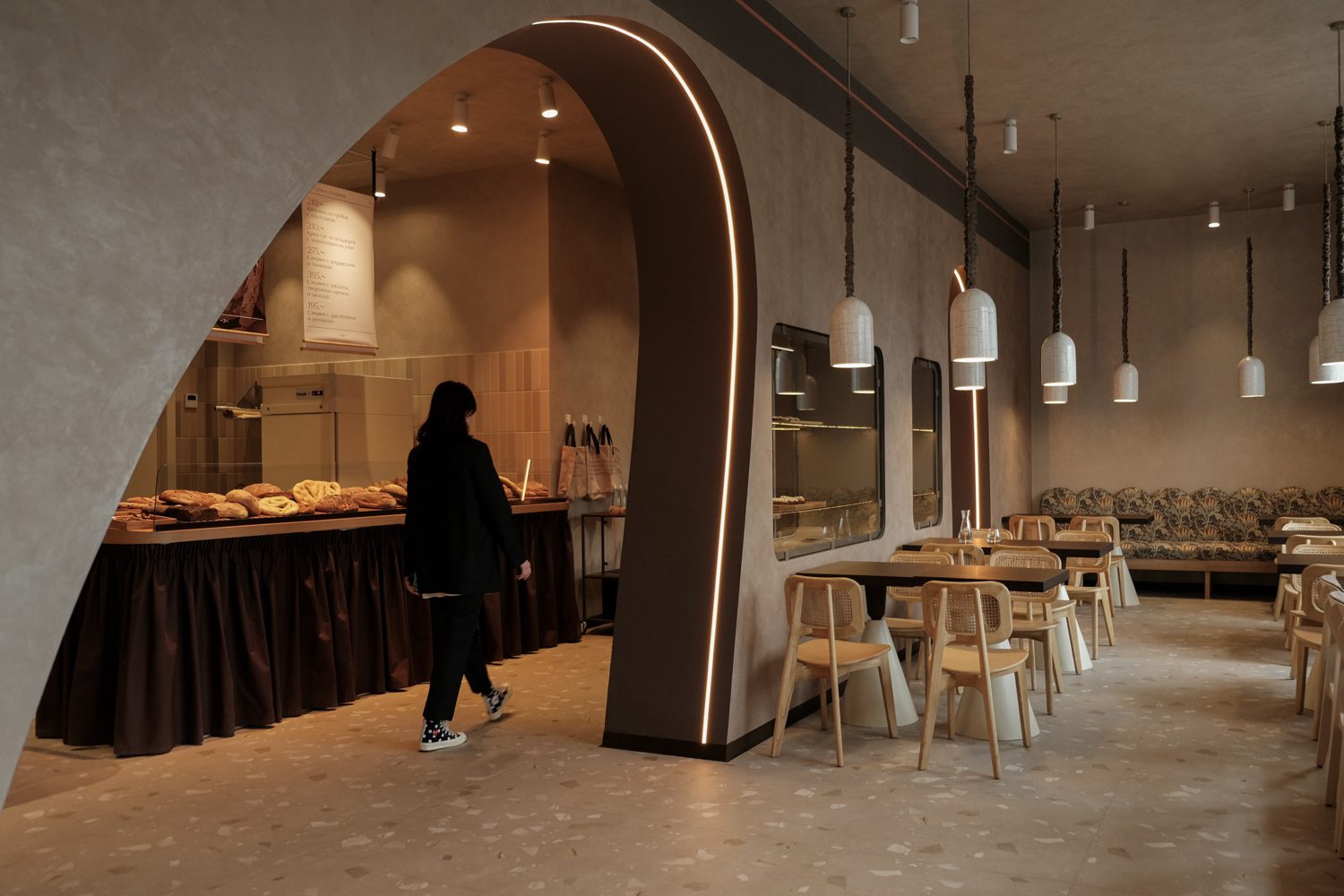This detailed photograph captures the inviting interior of a dimly lit restaurant or bakery with rustic stone-styled walls and a seamless light brown, speckled floor. The left side features numerous unoccupied wooden tables and chairs with wicker backs, their conical feet adding a touch of elegance. Overhead, delicate white conical light shades hang from the ceiling, casting a cozy glow. Central to the image is a light brownish-gray wall separating the dining area from the bakery showcase, where small windows display enticing pastries on racks. On the left, a large arched opening reveals another room with a sumptuously arranged pastry table, scattered with various breads, and a blurred menu above. A solitary woman in a black outfit with white shoes walks away, her long hair trailing behind, adding a human element to this serene scene.